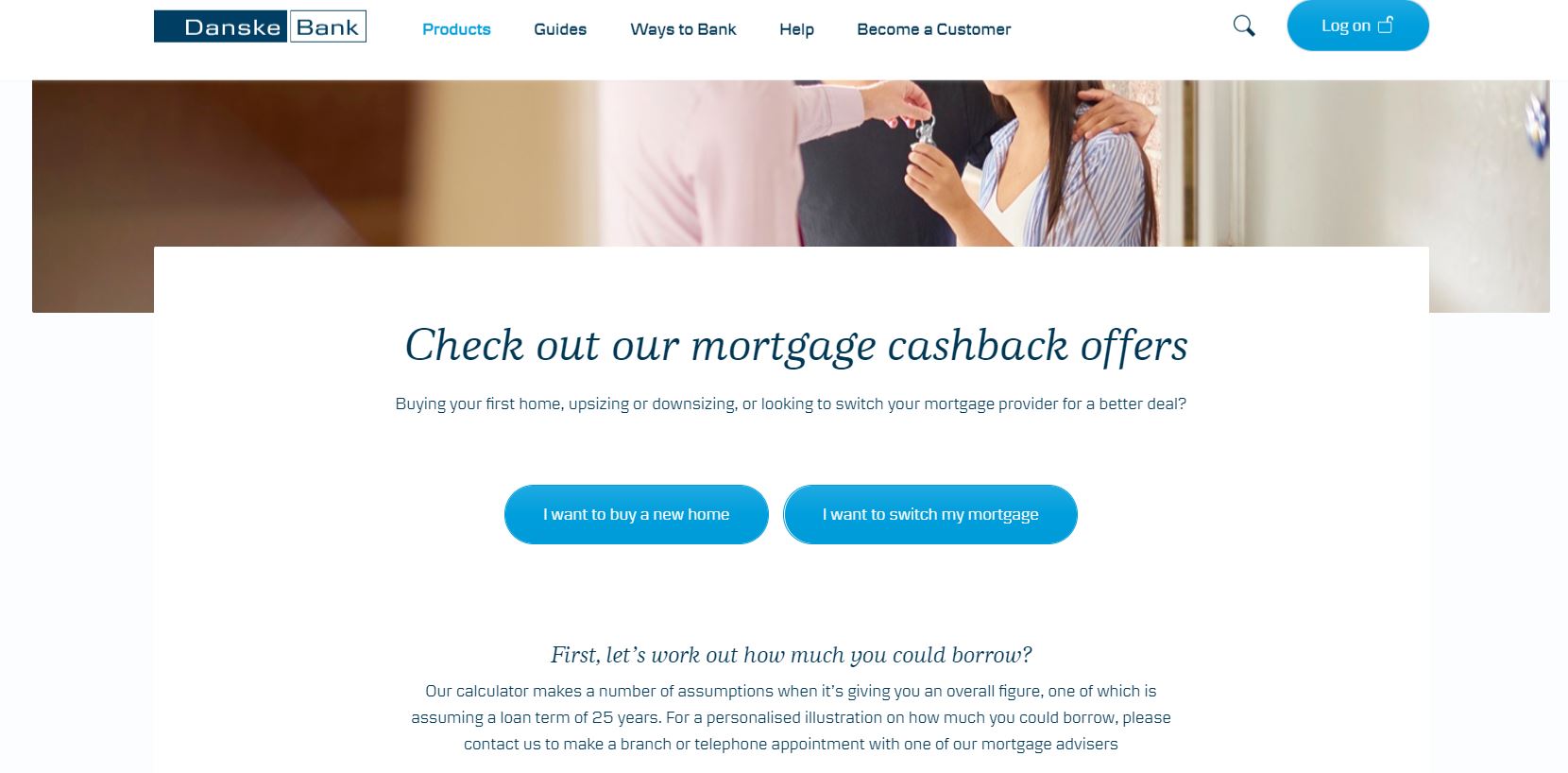This is a detailed caption of the Danske Bank webpage featuring their mortgage services. The webpage prominently displays a message inviting potential clients to explore Danske Bank's mortgage cashback offers. It caters to individuals who are either buying their first home, upgrading, or downsizing. The central section emphasizes the importance of determining borrowing capacity with the text: "First, let's work out how much you can borrow."

At the top, the navigation bar includes options for "Products," "Guides," "Ways to Bank," and a pathway to become a customer. Features such as a search function and a logout button are also visible. The imagery places a significant focus on homeownership, highlighted by a visual of one person handing a house key to another, symbolizing the transition to owning a new home.

Danske Bank, based in Denmark, is providing comprehensive information on mortgage plans, cashback offers, and more. The page serves as a gateway for users to delve deeper into the bank's mortgage options while also implying a range of other financial services accessible through the bank's navigation menu.